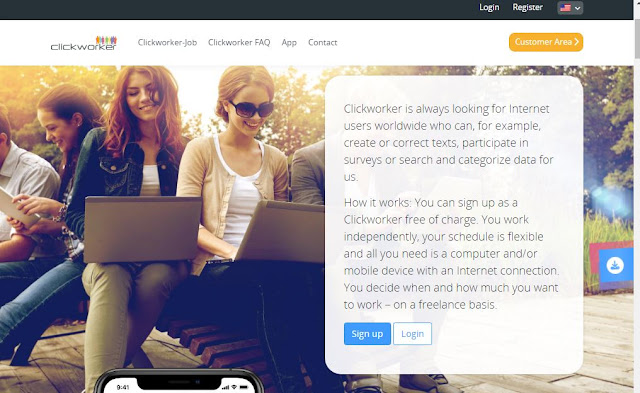This image is a screen capture of the ClickWorker website. At the top of the page, there is a gray bar in the upper right-hand corner, featuring an American flag with a downward arrow indicating a drop-down menu for selecting different languages or locations. To the right of this, there are options labeled "Register" and "Log In."

Below this gray bar, a white navigation bar spans the width of the page. On the left side of this bar is the ClickWorker logo, followed by buttons labeled "ClickWorker-Job," "ClickWorker-Fact," "App," and "Contact." On the far right side of the navigation bar, a yellow button labeled "Customer Area" is accompanied by a right-pointing arrow.

The main section of the page features a background image showing people working on laptops outdoors in a park-like setting with trees and sunlight. Five individuals are visible, though only three of their faces can be seen clearly; the others are partially cut off at the edges. The scene exudes a sense of casual productivity and community.

Overlaid on this background image is a white text box describing ClickWorker's mission. The text reads: "ClickWorker is always looking for internet users worldwide who can, for example, create or correct text, participate in surveys, or search and categorize data for us. How it works: you sign up as a ClickWorker free of charge. You work independently. Your schedule is flexible, and all you need is a computer or mobile device with internet connection. You decide when and how much you want to work on a freelance basis."

At the bottom of this text box are two buttons for user action: a blue "Sign Up" button and a white "Log In" button.